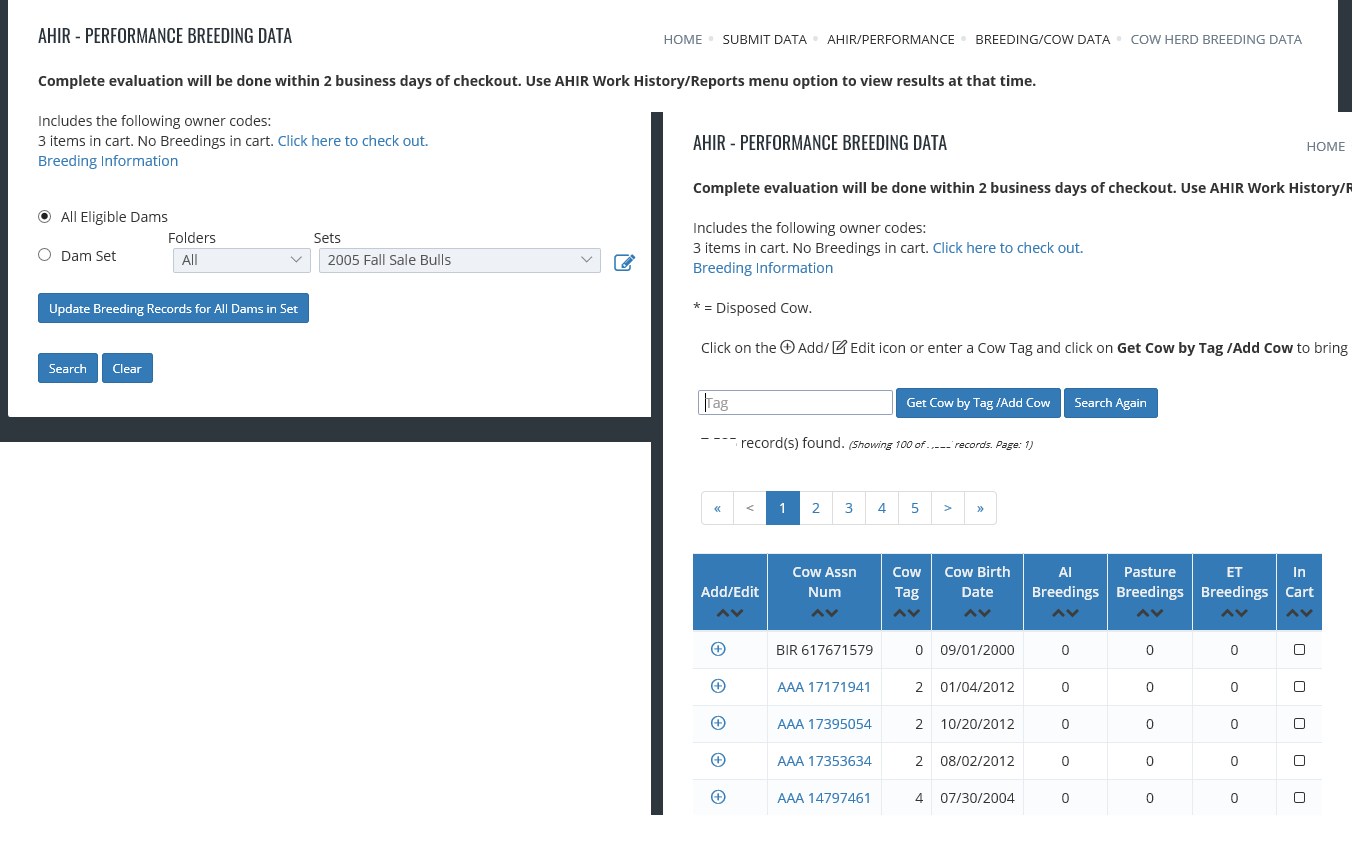Two screenshots of different sections of a website have been merged together against a white background. Each section is enclosed by a black bezel, creating a shadow effect.

### Left Section:
- **Header Text:** 
  - In bold black text: "AHIR - PERFORMANCE BREEDING DATA."
  - Below in another bold line: "COMPLETE EVALUATION WILL BE DONE WITHIN TWO BUSINESS DAYS OF CHECKOUT. USE AHIR WORK HISTORY/REPORTS MENU OPTION TO VIEW RESULTS AT THAT TIME."
- **Buttons and Links:** 
  - A sequence of grey, clickable buttons in all caps: "HOME," "SUBMIT DATA," "AHIR/PERFORMANCE," "BREEDING DATA," "COW HERD BREEDING DATA."
- **Information and Interaction:**
  - "INCLUDES THE FOLLOWING OWNER CODES, THREE ITEMS IN CART, NO BREEDINGS IN CART," in black text.
  - A blue hyperlink: "CLICK HERE TO CHECKOUT."
  - Another blue hyperlink: "BREEDING INFORMATION."
  - Selected radio button labeled "ALL ELIGIBLE DAMS," indicating selection by a black circle within.
  - Unselected radio button labeled "DAM SET."
  - A heading labeled "FOLDERS" followed by a dark grey dropdown rectangle with entries "ALL" and "SETS."
  - Dropdown entries: "2005 FALL SALE BULLS."
  - Icon: A blue-bordered paper with a blue pencil over it.
  - Dark blue rectangle with white text: "UPDATE BREEDING RECORDS FOR ALL DAMS IN SET."
  - Buttons labeled "SEARCH" and "CLEAR."

### Right Section:
- **Instructions and Buttons:**
  - Text: "ASTERISK = DISPOSED COW." 
  - Instruction to "CLICK ON THE CIRCLE OR THE PLUS ADD/EDIT ICON."
  - Bold text: "ENTER A COW TAG AND CLICK ON 'GET COW BY TAG/ADD COW'."
  - Search bar with grey text "TAG" and a blinking cursor.
  - Two dark blue rectangles:
    - The first, larger, with white text: "GET COW BY TAG/ADD COW."
    - The second with "SEARCH" in white text.
- **Pagination and Records:**
  - Italicized text: "(100 RECORDS FOUND)"
  - Label: "RECORDS PAGE 1"
  - Pagination: 
    - Dark blue rectangle indicating the current selection: "1" in white.
    - Next page options: "2, 3, 4, 5" in blue text within white rectangles.
    - Blue arrows: Double arrows for beginning and end of the pages, single arrows for next and previous pages.
- **Details of Listed Cows:**
  - Each listed cow displays:
    - Number
    - Cow Tag
    - Birth Date
    - Breeding Procedure
    - Pasture Breeding
    - ET Breeding
    - End Cart